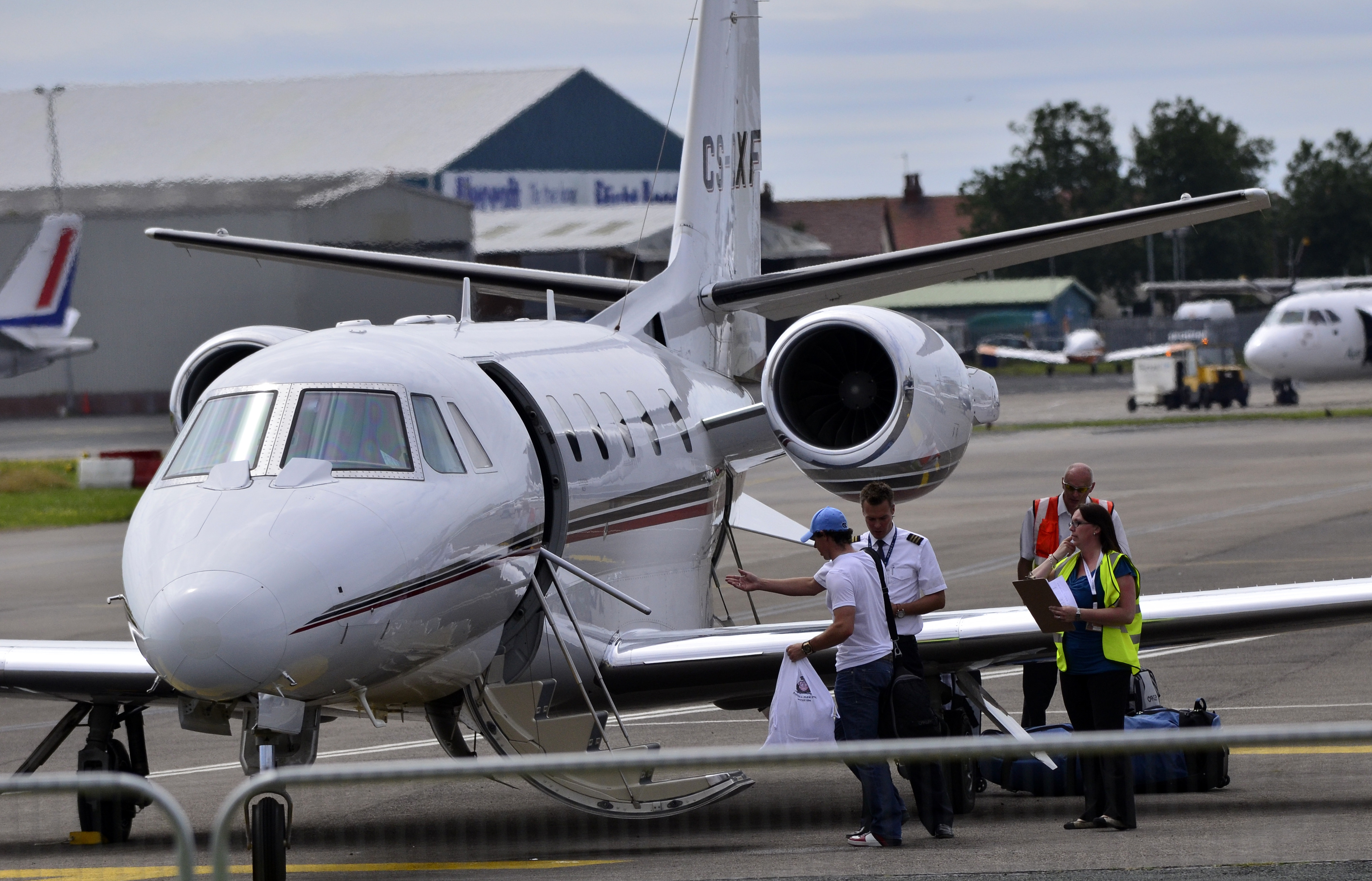The image captures a smaller, likely private jet positioned on a tarmac at a private airport. The aircraft is largely white, adorned with black, gray, and red stripes running along its body from nose to tail. The plane's orientation reveals part of its side and front, angled in a seven o'clock direction. It features five visible rows of windows on its side, two turbines, standard wings, and a tail with fins.

On the ground beside the jet, there is a group of individuals. A man wearing a blue baseball cap, a white t-shirt, and blue jeans is seen boarding the jet carrying a plastic bag and a duffel bag slung over his shoulder. Nearby, a woman with white hair, clad in a neon yellow vest and holding a clipboard, is positioned next to a man in an orange vest. Another man, presumed to be the pilot, stands near the plane's wing in a white shirt with shoulder patches. The scene includes additional background details: an array of buildings, some trees, and other planes visible at a distance, further suggesting a bustling airport environment.